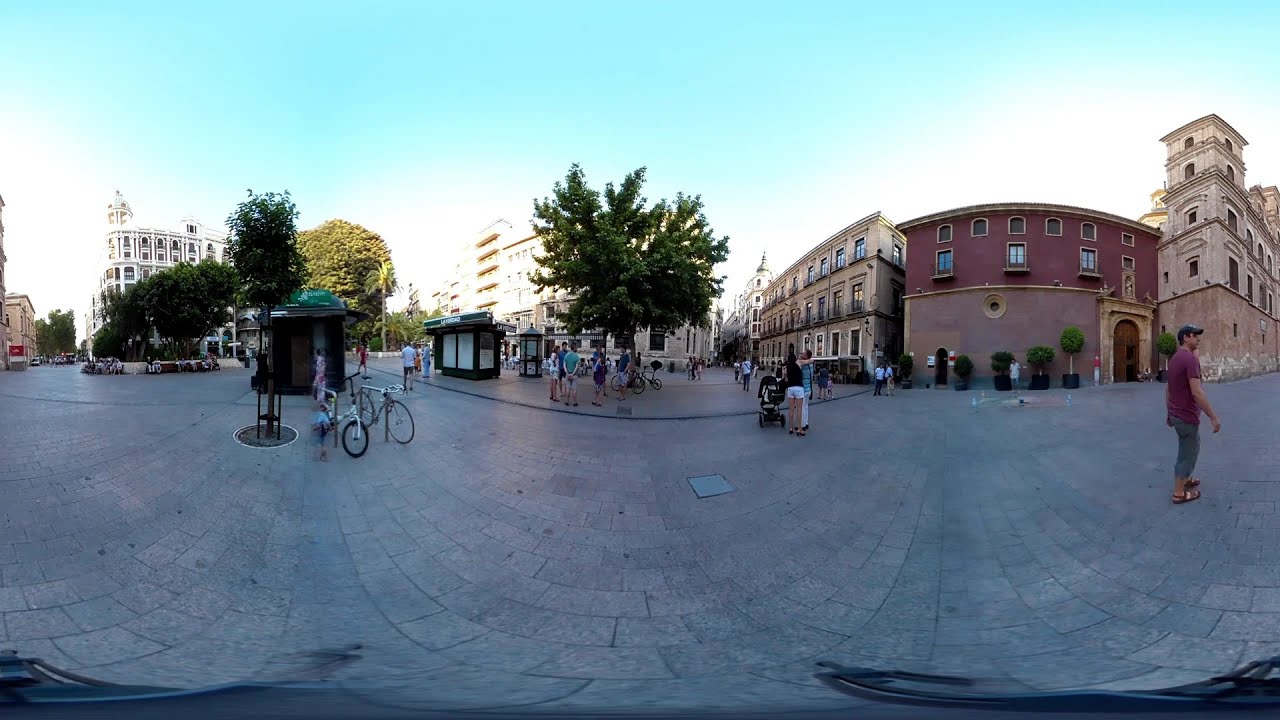The image captures a charming city center bathed in beautiful weather, likely in the afternoon. The sky is a stunning blue with occasional clouds near the horizon. The scene features a blend of historical-looking buildings in shades of white, red, and brown, encircling a spacious, tiled walking area. The ground consists of small square tiles in a brick-and-cement design, hinting at an old-world, possibly European or Asian, ambiance. Among the greenery of lush trees, people dressed in summer clothing leisurely stroll around, with some pushing strollers and others standing or walking in small groups. Bicycles are parked intermittently along the sidewalks, and bus stops are visible. 

In the foreground, towards the right edge of the image, a man wearing a grey hat, dark red t-shirt, grey pants, and flip-flops strides to the right, adding a focal point to the scene. Though not overly crowded, there are definitely over ten people dispersed throughout, some of whom appear to be tourists, adding to the bustling yet relaxed atmosphere. This picturesque city center offers a vivid snapshot of everyday life and leisurely activities under a pleasant sky with the sun positioned moderately low, casting a soft, warm light over the scene.